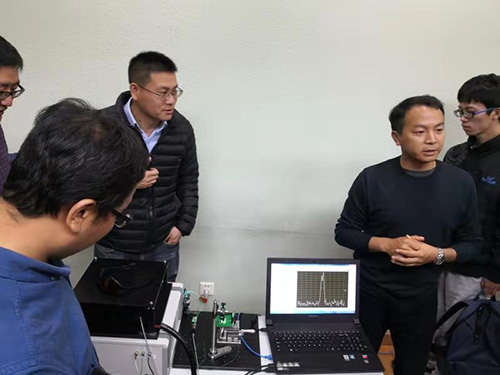In this outdoor photograph, five individuals are positioned in front of a clean, white or light gray wall devoid of any decorations such as paintings, drawings, or bookshelves. Each person is standing, although none are fully visible. 

On the far right, a person with dark hair and glasses is partially visible, showing just a bit of his head and part of his face. To the lower left, another individual, mostly turned away from the camera, is wearing a blue shirt and glasses, with dark hair visible from the back. In the background on the left side, a man sporting short dark hair and glasses gazes to the right, dressed in a blue shirt with a black jacket over it. 

On the right side of the image, there are two more individuals. One appears to be of Asian descent, with dark hair, wearing a black sweatshirt and a watch on his left wrist. Beside him stands a younger man with dark hair and glasses, wearing a dark top and seemingly holding a backpack. They are positioned near a table that holds a laptop with its screen on, displaying a graph, along with other computer components.